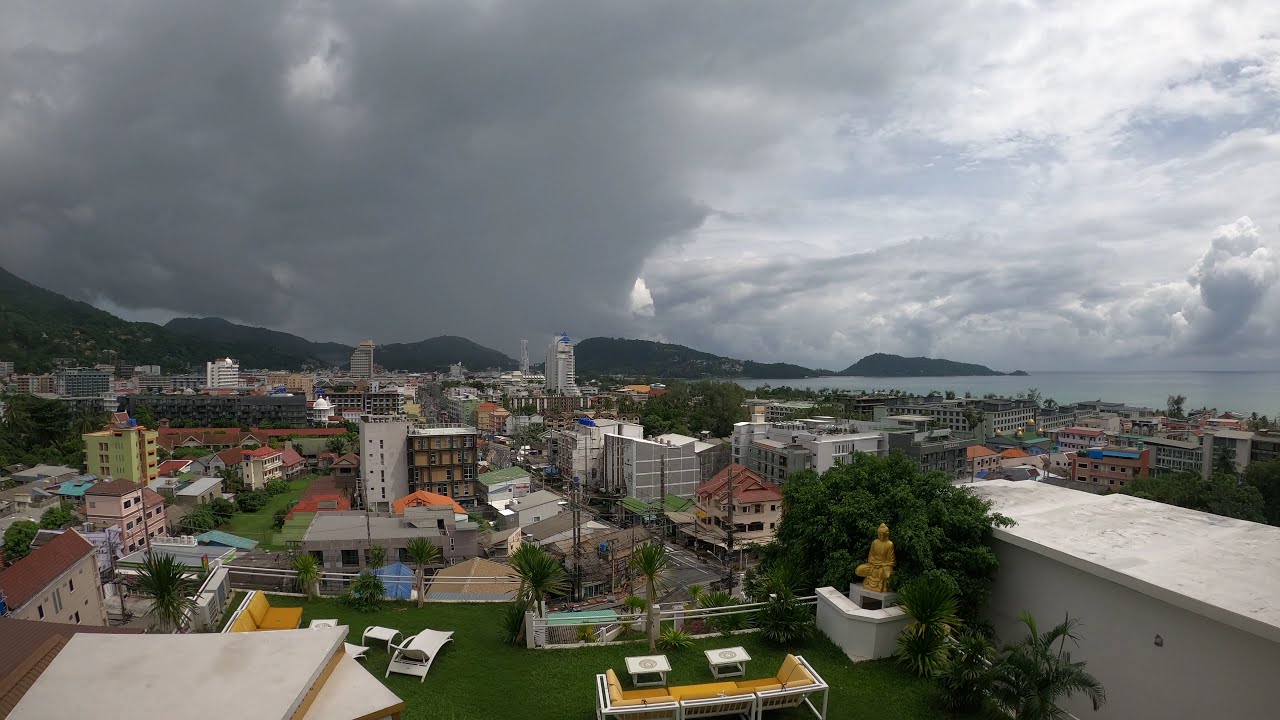This image, taken from a high vantage point atop a building, captures a detailed and vibrant urban landscape. On the building's roof, there's a striking setup featuring green artificial grass, two couches adorned with yellow cushions, two white lounge chairs, and several small white chairs, creating a cozy seating area. Nearby, a golden statue of Buddha adds a unique touch. Just over the fence of the rooftop, a street is barely visible. 

The panorama reveals a bustling residential area punctuated by numerous multi-story buildings in varied colors including yellow, brown, tan, and white. To the left of the image stands a yellow residential building, and centrally located is a brown building with many windows. Adding to the scene's dynamics, there are lots of palm trees scattered throughout, with prominent ones on the left and bottom center. The backdrop features colossal, lush green mountains and further in the distance to the right, the expansive blue ocean glimmers. 

The skyline is dramatic, dominated by heavy, dark clouds that obscure much of the midday sun, casting a dim light over the scene. This moody atmosphere underscores the enormous scale of the mountains and the serenity of the coastline, possibly indicating a locale like New Zealand. The assortment of buildings—ranging from office high-rises to colorful and tall residential complexes—contrasts sharply against the natural beauty in the distance, creating a compelling and richly detailed urban vista.